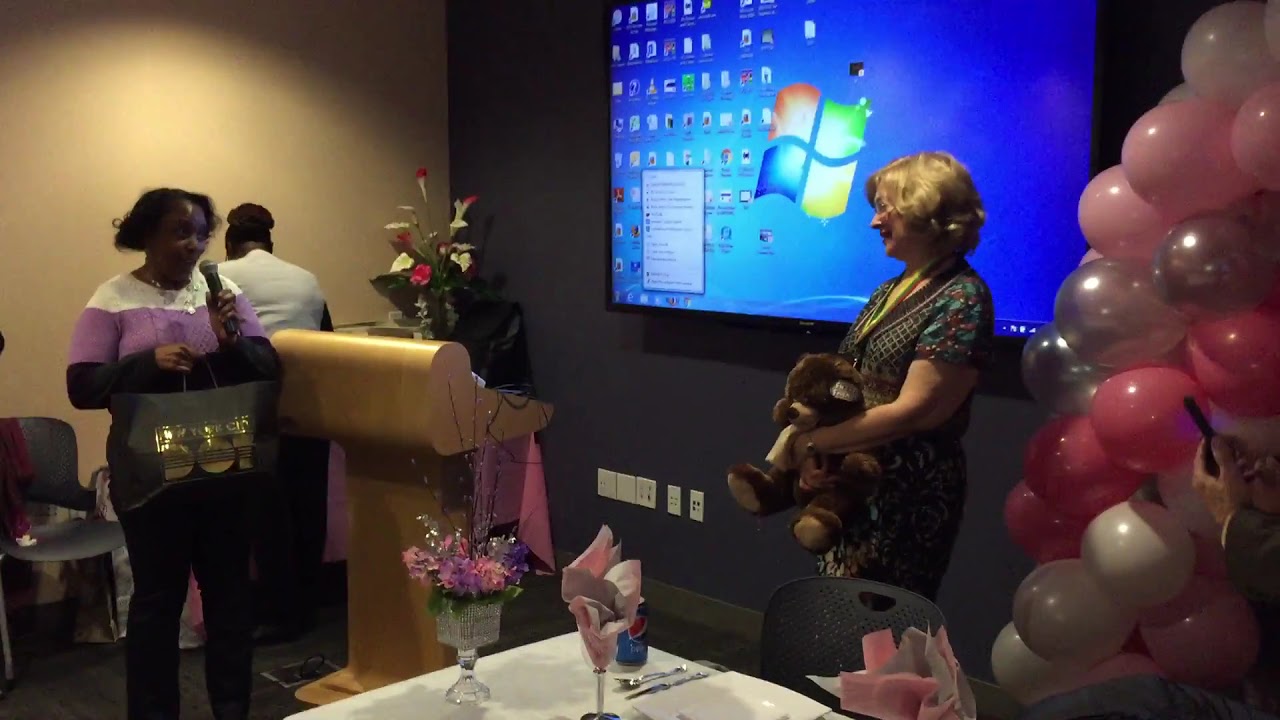In this vibrant indoor office party scene, three main attendees are captured amidst lively decorations and a large presentation screen displaying a typical computer desktop with icons and the Windows logo. To the left, a woman with brown hair, dressed in a purple and white shirt, holds a black gift bag and a microphone, seemingly addressing the attendees. To her right, a blonde-haired woman, wearing a blouse, stands smiling while holding a brown teddy bear. They appear to be the central focus of an animated interaction. Surrounding them, colorful pink, silver, and white balloons add a festive touch, while a table adorned with flowers, a Pepsi can, and utensils sits at the foreground. In the background, a man's back is visible, adding depth to the busy, celebratory atmosphere, and to the far side, the hands of another individual holding a phone can be seen. The scene suggests a celebratory event, likely a going-away or congratulatory party, filled with warmth and camaraderie.